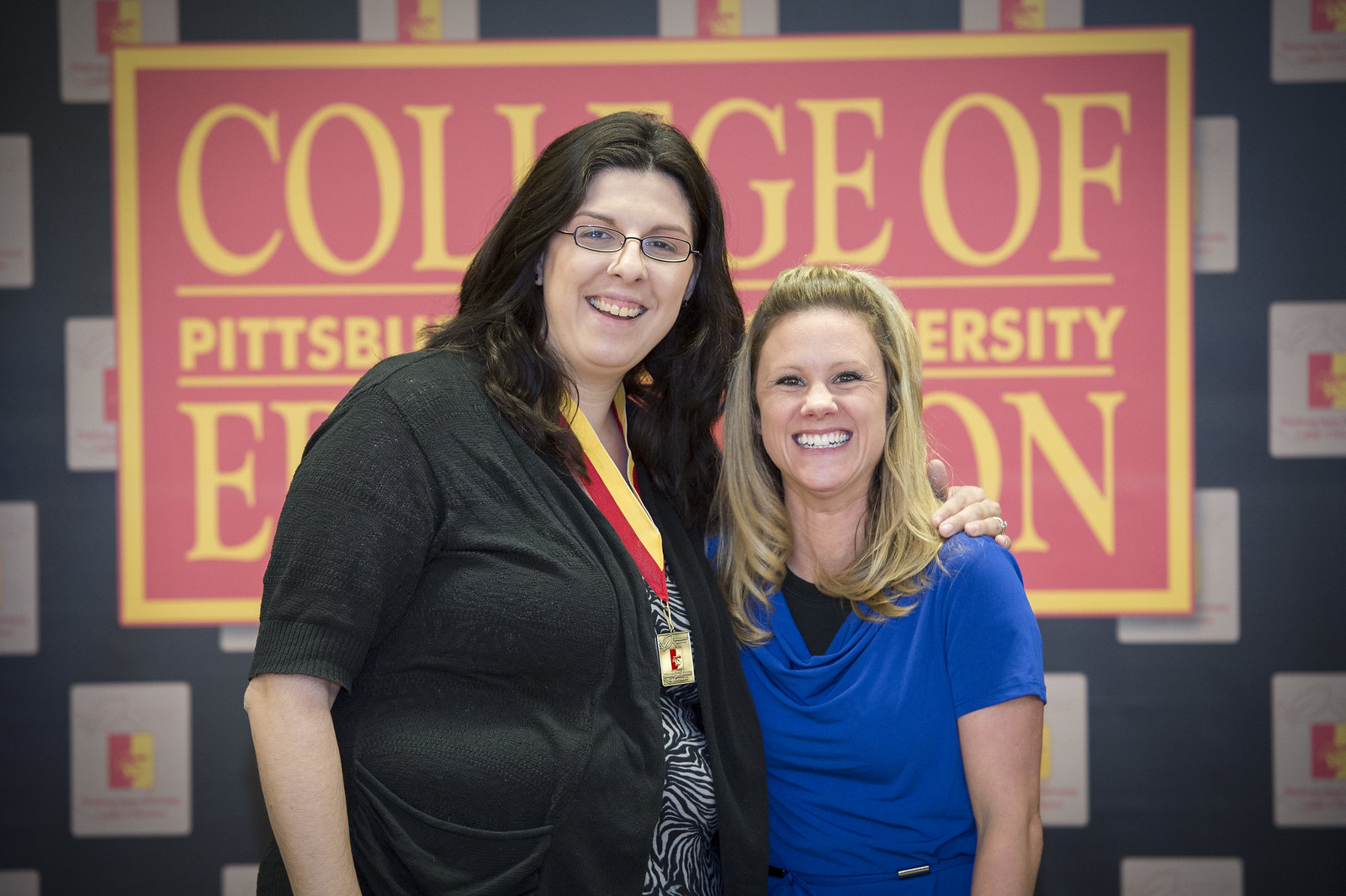In this vibrant university event picture, two women are posing and smiling at the camera against a backdrop that features a dark blue wall adorned with white squares and artistic images of gorilla faces in red and yellow hues. The wall is partially covered by a prominent red rectangle outlined in gold, which bears the partially obscured text "College of Pittsburgh University." Both women are dressed in complementary colors that echo the event's theme. The woman on the left, with long dark brown hair and black-framed glasses, is wearing a black cardigan over a black and white zebra-print shirt, accessorized with a red and gold award ribbon around her neck. The woman on the right, slightly smaller in stature, has long blonde hair and is wearing a blue shirt over what appears to be a black top. Both women are beaming with joy, evidently enjoying the celebration.